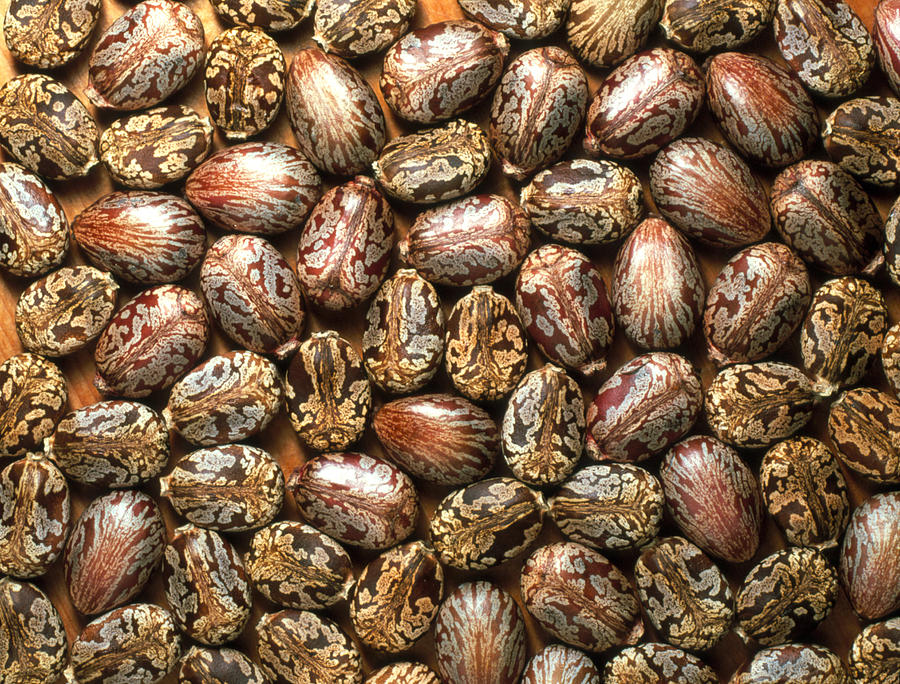The image features an almost square photograph, slightly oriented in landscape format, set against a medium-shaded wood background that subtly peeks through. Spread across this wooden surface are approximately 50 shiny, oval-shaped objects whose true size is indeterminate due to a lack of comparison. These objects display a plethora of intricate, ornate designs and come in various hues including shades of browns, golds, and hints of bluish-gray. The designs are detailed, with patterns varying from a whiter color on rustier brown objects to a creamy tan on darker browns. Though they could be mistaken for bugs, coffee beans, or even gemstones, their exact nature remains ambiguous. They lie flat, seemingly scattered or haphazardly spread out, partly overlapping yet leaving some gaps between them. The framing of the image cuts off part of these objects along the edges, adding to the enigmatic visual.